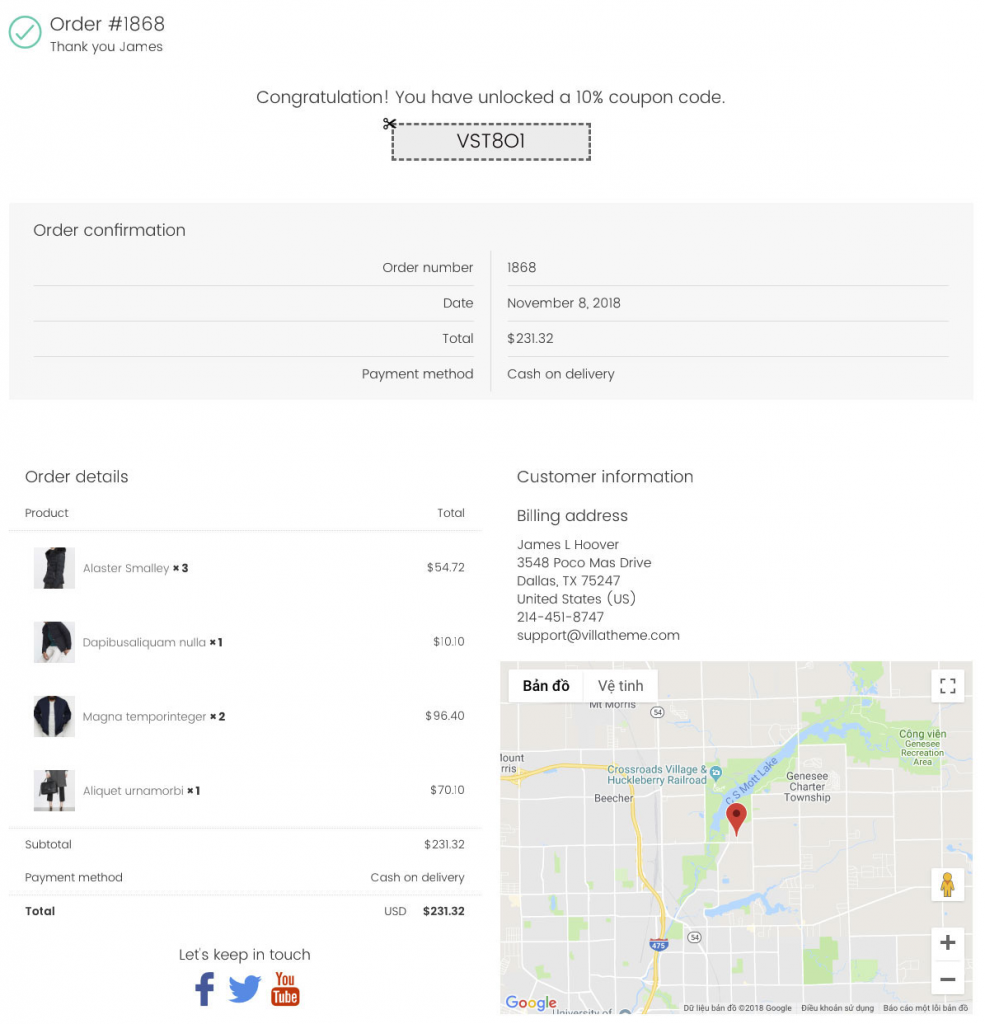The image depicts an invoice with detailed transaction information. At the top left, there's a green checkmark and the label "Order Number: 1868." Below this, there's a message thanking a customer named James. 

In the center of the invoice, there's a prominent congratulatory message stating, "Congratulations! You have unlocked a 10% coupon code," displayed in black text on a white background. Below this, a grey, perforated bar contains the actual coupon code.

Underneath the coupon section, the invoice provides the order confirmation details, including the order number and the date, November 8th, 2018. The total amount for the order is highlighted as $231.32, with the payment method specified as cash on delivery.

Moving on to the order specifics, it lists four products without detailed descriptions, contributing to the total sum of $231.32. Further information includes the customer's billing address: James L. Hoover, 3548 Pacomas Drive, Dallas, Texas, 75247, United States. Contact details such as a telephone number and support email (support@villatheme.com) are also provided. A small section marks the location on a map.

The invoice wraps up with all these specifics clearly laid out for verification and record-keeping.